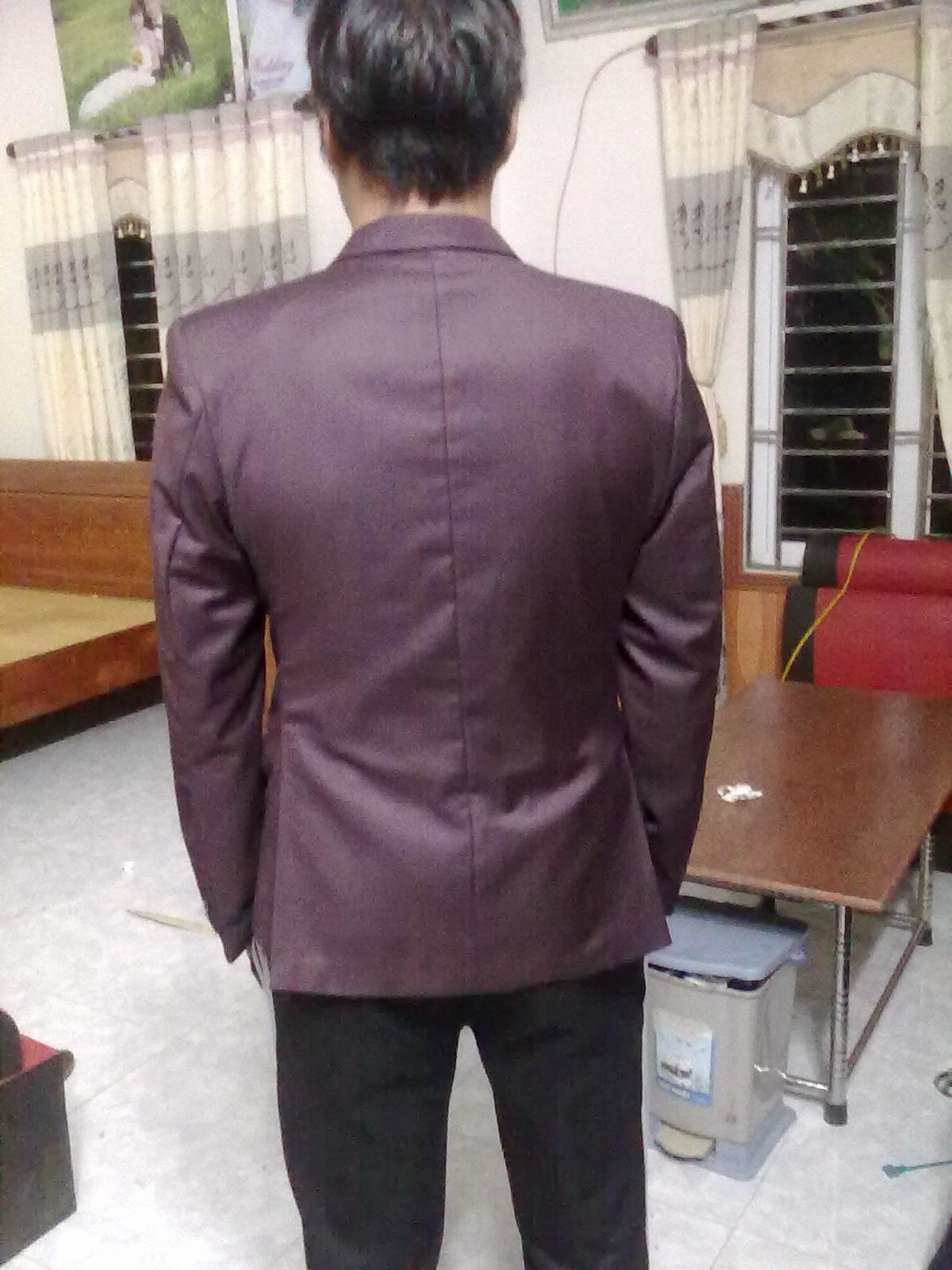This color photograph captures the back of a man standing indoors, seen from the knees up. He is dressed in formal wear, sporting black slacks and a dark purple blazer, with short black hair visible. The setting features gray tiled flooring and white walls adorned with a canvas photograph of a bride and groom sitting in a green field, positioned in the upper left corner. The room has windows on either side, covered by beige curtains. In front of the man is a small trash can and a brown table, contributing to the casual ambiance of the space.